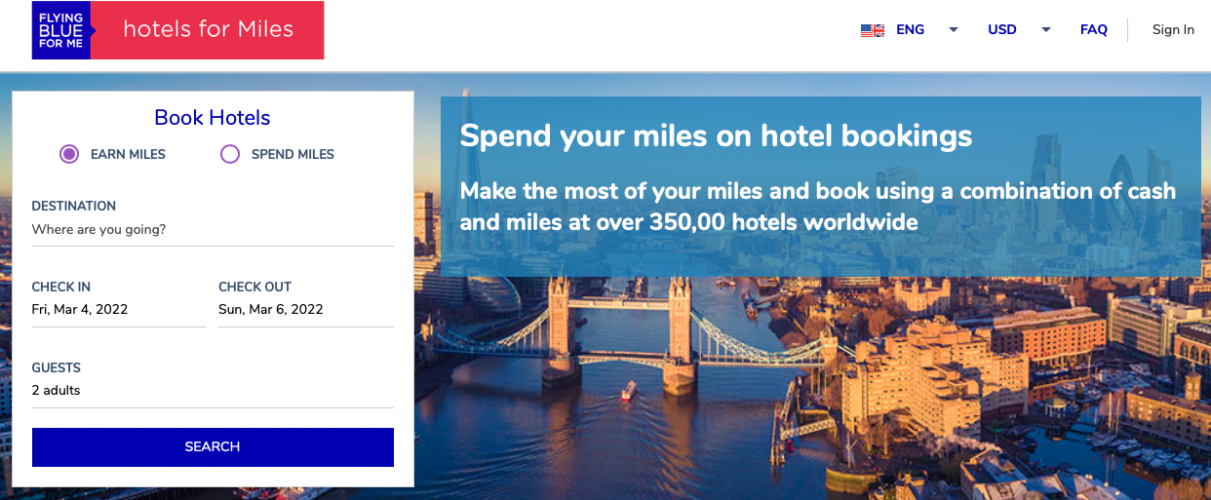The image showcases a detailed advertisement web page for booking hotels. The primary section prominently features various types of buildings, indicating different hotel options available for purchase. Users are prompted to enter their travel details, including destinations, arrival and departure dates, and the number of guests.

At the top of the page, there is a navigation bar with multiple icons that facilitate accessing additional information. These icons likely provide functionalities such as changing the language, converting currency, or retrieving more detailed sections of the website. 

There is also a dedicated help section, where users can find answers to frequently asked questions or request further assistance. 

Additionally, a login area is visible, allowing users to enter their personal information and access their accounts. This feature offers a personalized browsing experience, enabling users to manage their bookings and preferences effectively.

Overall, the web page is designed to be user-friendly and comprehensive, ensuring a smooth hotel booking experience.